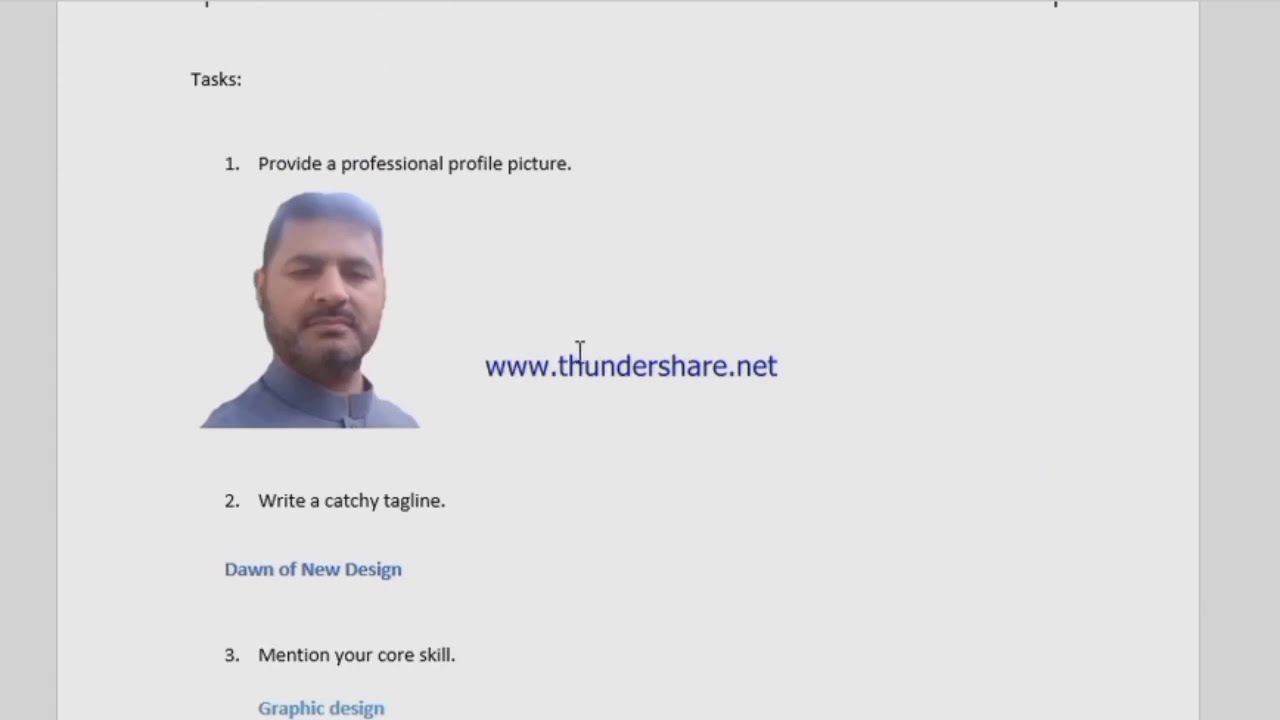The image is a screenshot of a Word document that serves as a guide for crafting a social media profile. The document's background is predominantly white, framed by darker gray margins on both the far left and far right sides. Prominently placed in the upper left corner is the header "Tasks" in black print, followed by a numbered list. 

The first item on the list reads "1. Provide a professional profile picture," beneath which is a photo of a man with Caucasian skin, short brown hair, thick brown eyebrows, a straight nose, heavy-lidded eyes, a mustache, and a close-shaven beard. He is wearing a high-collared light blue dress shirt. To the right of his photo is the website link "www.thundershare.net" in blue text.

Item two on the list states "2. Write a catchy tagline," followed by the phrase "dawn of a new design" in blue text. The third item reads "3. Mention your core skill," beneath which the text "graphic design" appears in blue. The remainder of the document is blank, with the instructional text and image creating a visually structured yet minimalistic layout.